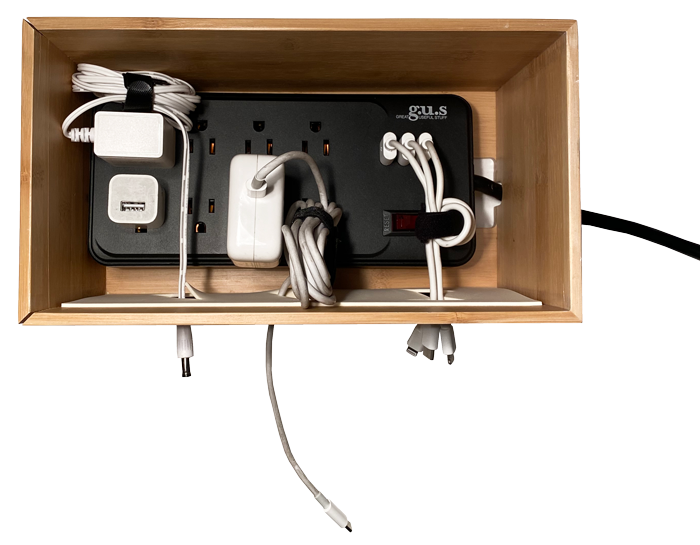This top-down, bird's-eye photograph captures a large, black power strip neatly enclosed inside a wooden box with custom-made holes for cord management. The power strip features eight standard outlets and three USB ports. All three USB ports are occupied by white cables, each extending out of the box without being connected to any devices on the other end. Among the standard outlets, three are occupied by iPhone chargers, also with their ends untethered, unplugged from any devices. Another charger, which appears to be for a MacBook, is plugged into the power strip, its cord neatly tied. Additionally, there is a yet-to-be-identified charger with a long, tied-up cord. In total, six cords are plugged into the power strip, with the wooden box providing a tidy and organized setup for managing multiple electronics.